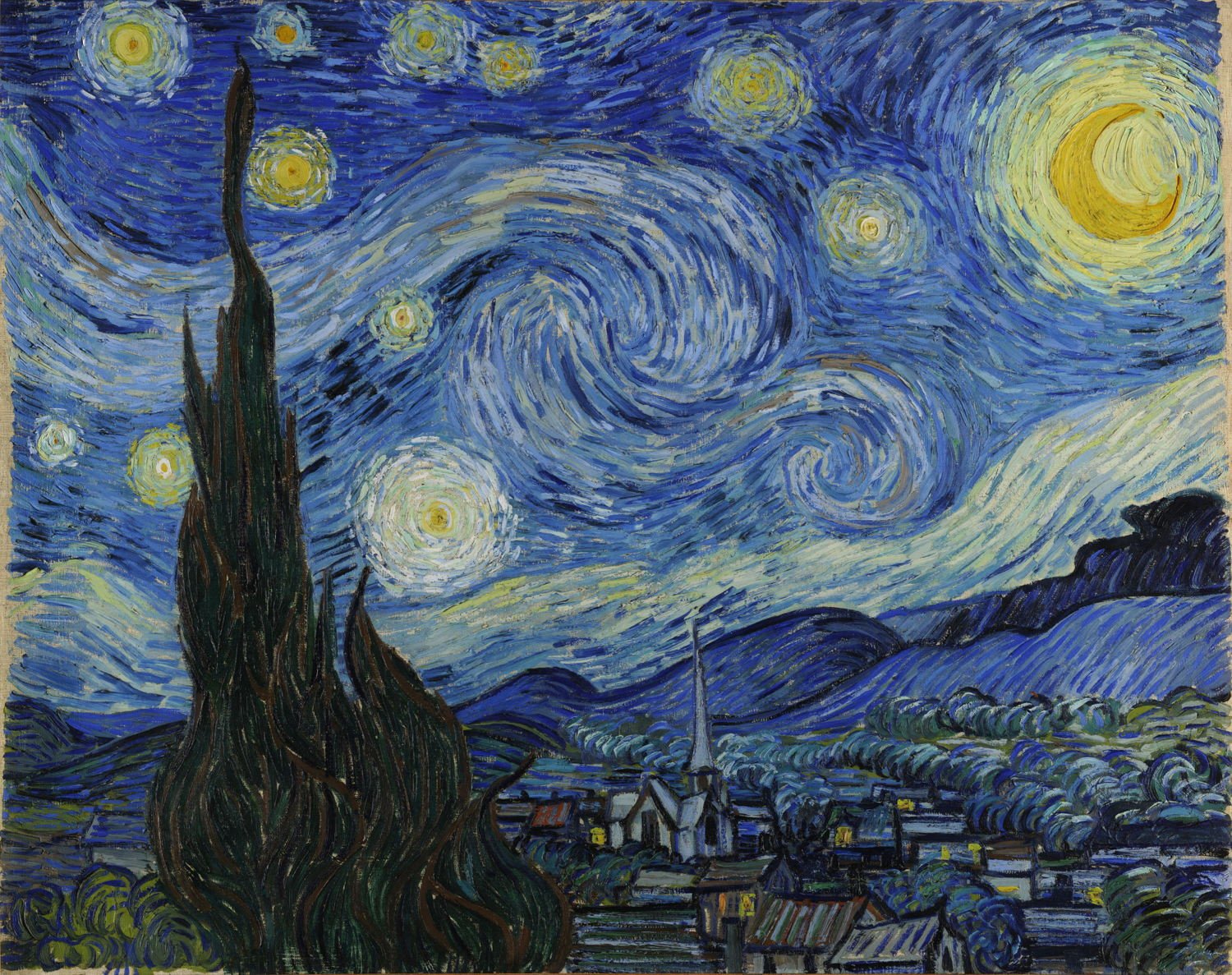This painting appears to be a famous work by Vincent van Gogh, commonly known as "The Starry Night." Dominating the canvas is a mesmerizing night sky filled with dynamic, swirling patterns. The moon, depicted as a crescent, radiates light encircled by luminescent swirls. Numerous stars are scattered across the sky, each encircled by its own halo of light. A wavy band of wind currents flows horizontally across the sky, adding to the sense of movement.

Beneath the celestial display lies a quaint village, which could be French or Dutch in origin. The village comprises simple, flat-roofed houses, each with distinct striped patterns on their roofs, adding texture and interest. To the lower left of the composition stands a prominent cypress tree, its dark, elongated form contrasting sharply with the vibrant sky.

Central to the village is a church, distinguished by its tall, thin spire that reaches towards the heavens. Behind the village, a series of gently rising hills and mountains extend from left to right, framing the scene in the background.

This iconic painting is celebrated worldwide and is undoubtedly displayed in a renowned museum, capturing the imagination of countless admirers.